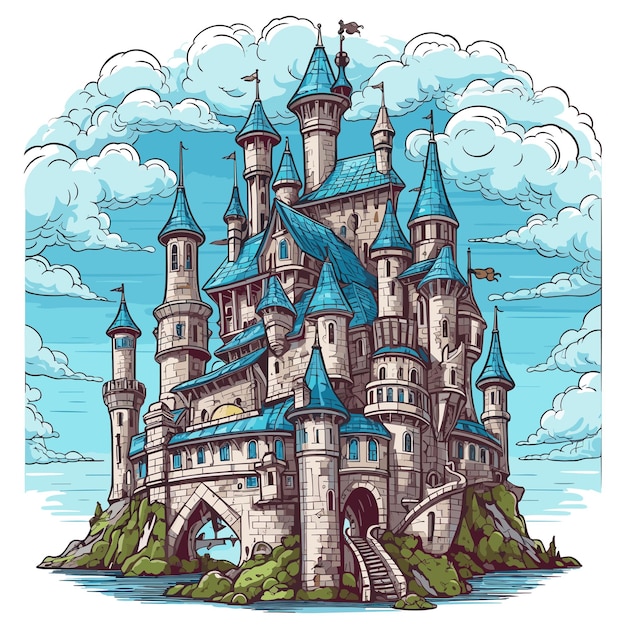This whimsical, digitally colored and inked illustration depicts a fantastical, medieval-style stone castle perched on a small, lush green island surrounded by a serene body of water. The castle's intricate architecture features numerous circular towers and turrets, each topped with pointy turquoise roofs, some adorned with flags. The walls of the castle exhibit a blend of beige, brown, and light gray stone, with several water entranceways hinted at by arches at its base. A sturdy stone stairway descends directly into the water, emphasizing the castle's island setting. Framing the castle are fluffy white and light blue clouds that arc gracefully around it, set against a backdrop of a vividly blue sky. The detailed, cartoonish nature of the illustration, highlighted by solid ink lines, evokes a sense of whimsy reminiscent of classic fairytale imagery, much like the iconic Disney castle. The absence of people in the scene enhances the mystical and serene atmosphere of this enchanting island fortress.